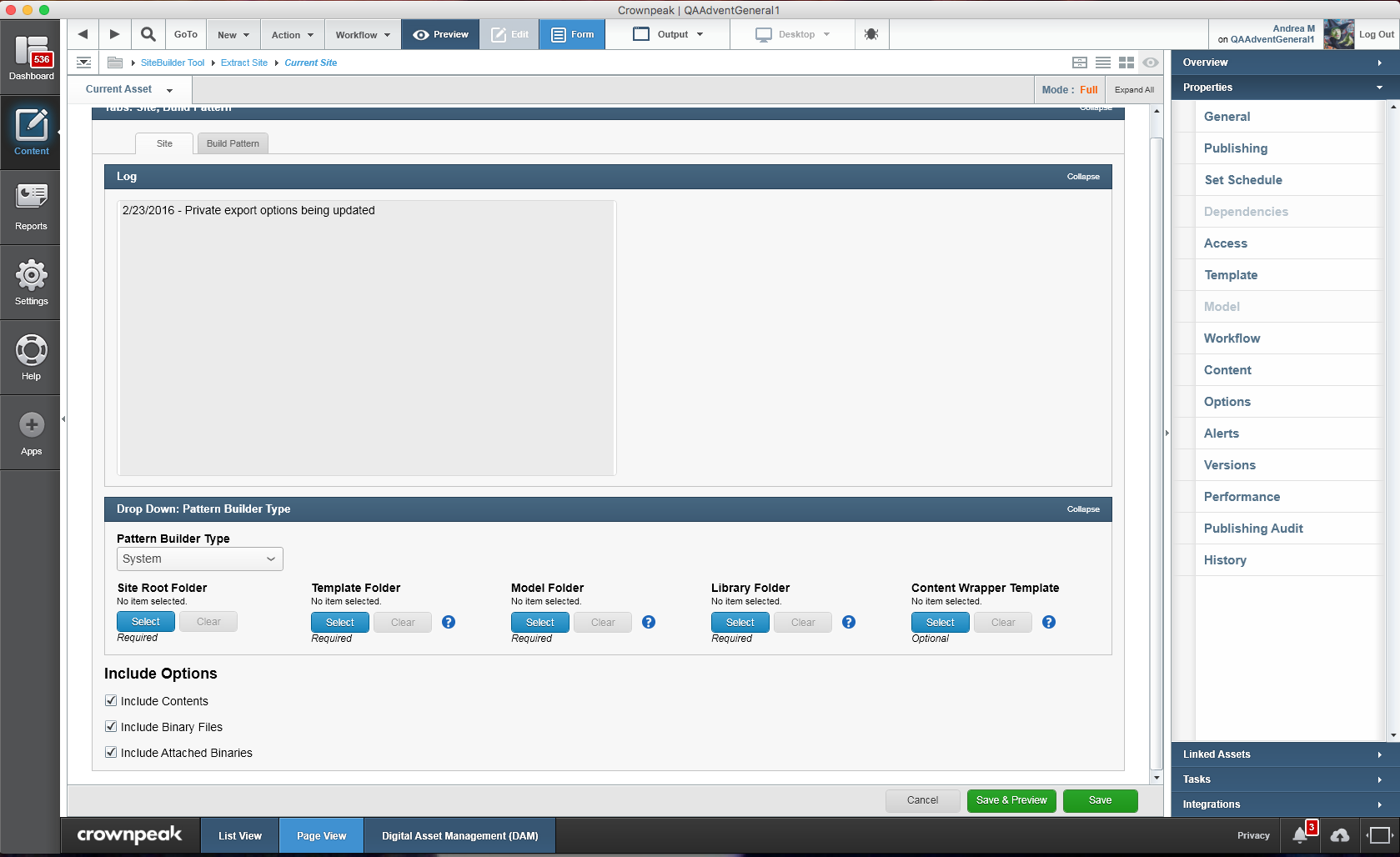The image appears to be a screenshot of a computer interface, likely a settings or configuration menu for a software application. On the left side of the interface, there is a white pen icon inside a square, situated above a white piece of notebook paper. Below this, there is a white wheel icon labeled "Settings." Further down, a white and gray circle is labeled "Help." Beneath "Help," there is a gray circle with a plus sign inside it, labeled "Apps."

Moving down the interface, there is a clickable area with a downward arrow, preceded by the label "Pattern Builder Type" inside a section titled "System." The interface also displays various categories in black text: Site, Root Finder, Template Folder, Model Folder, Library Folder, and Content Wrapper Template.

At the bottom of the interface, there are two green buttons. One is labeled "Save," while the smaller button next to it saying "Save in Pictures." 

On the far right side of the interface, there are additional group options listed in blue text: General, Publishing, Set Schedule, Access, Template, Workflow, Content, Options, Alerts, Performance, and History. These categories suggest robust functionality and customizable settings within the software.